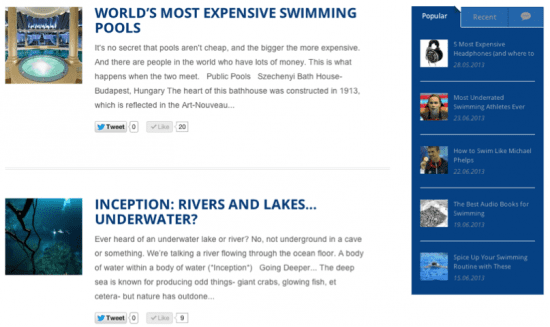A detailed caption for the given image could be formulated as follows:

---

Screenshot of a webpage titled "World's Most Expensive Swimming Pools." The main image features a luxurious circular pool surrounded by ornate pillars, reflecting early 20th-century Art Nouveau architecture, specifically the Széchenyi Bathhouse in Budapest, Hungary, which was constructed in 1913. The accompanying text highlights the opulence of certain swimming pools, emphasizing that extravagant pools are a result of combining wealth with elaborate design. 

Below this, an engaging section titled "Inception" describes the phenomenon of rivers and lakes that exist underwater, presenting an enigmatic narrative about these unique natural occurrences. However, the text abruptly ends, hinting at more intriguing content. The section features social media engagement options with a tweet button and a like count of 9.

To the side, the webpage features a "Popular" section displaying various headlines, including "The Five Most Expensive Headphones," alongside related images. A "Recent" section is also visible, providing the latest updates. At the bottom-right corner, a circular messaging icon with three dots on a blue background is prominent, ready for user interaction. The overall design of the webpage is clean, with a predominantly white background and black text.